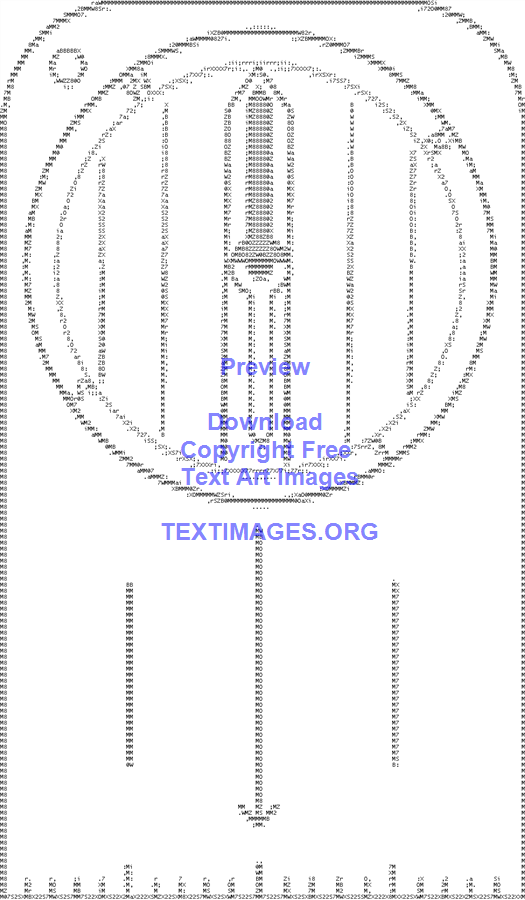The image showcases an intricate piece of text art that primarily depicts a compass. The design is mostly black and white, with the directional indicators—north, south, east, and west—clearly visible, forming a perfect circle. Inside this circle, there's a pointer that serves as the compass needle. The entire compass is situated within a larger, mostly rectangular area, though the top corners are gracefully rounded. Below the compass, a downward-pointing arrow is prominently displayed, flanked by a few vertical lines on either side.

Accompanying the visual elements, a watermark is overlaid in a purple font, reading, "Preview, download copyright-free text art images, textimages.org." The overall composition, while abstract, is meticulously crafted using text characters to form its geometric shapes, lending it a highly stylized and unique appearance.